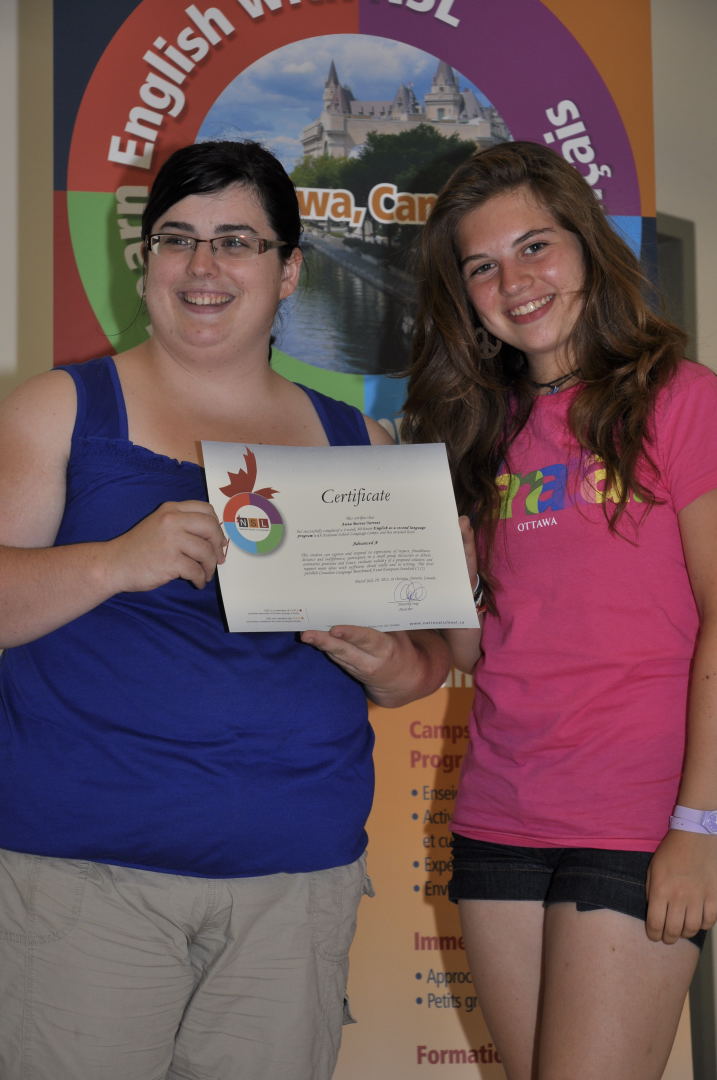In the image, two smiling women stand side by side, facing towards the camera, each holding a certificate. The woman on the left, who has dark almost-black hair either cut short or tied back in a ponytail, wears glasses, a blue tank top, and khaki pants. She holds her certificate with both hands in front of her. The woman on the right, with long brown hair cascading past her shoulders, is dressed in a pink t-shirt and black shorts, holding her certificate in one hand while the other rests neutrally by her side. Behind them towers a large, colorful sign featuring varied hues of red, blue, purple, orange, green, light blue, pink, light green, yellow, dark blue, grey, and black. The sign bears the words "Ottawa, Canada," along with an image of a river and a castle-like building. The certificates prominently display the word "Certificate," celebrating their achievement.